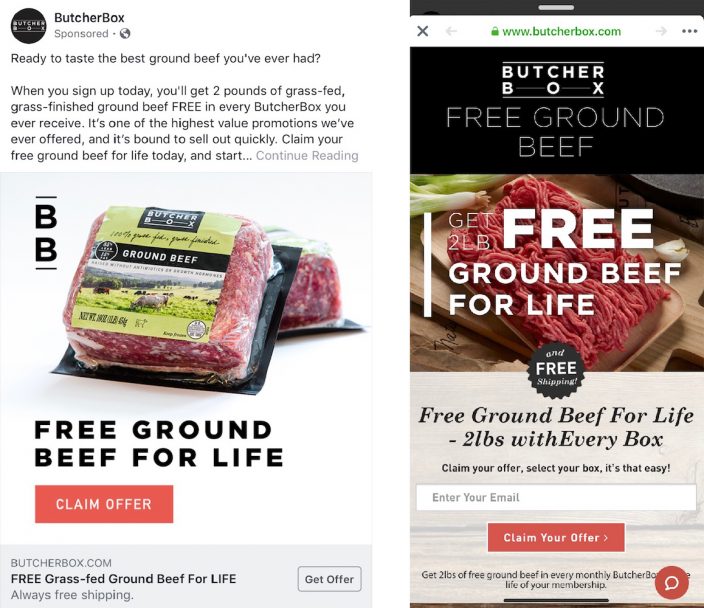The image is split into two panels, each providing information about a promotional offer from ButcherBox.

**Left Panel:**
At the top, a black circle prominently features the ButcherBox logo in white text. Surrounding the circle, the words "ButcherBox" are displayed again in white text against a black background. Below this, a gray print indicates the post is "sponsored."

The main content begins with a headline inviting viewers to "Taste the best ground beef you've ever had." Adjacent to this text, there's a graphic comprising the letters "BB" stacked creatively. The panel showcases various product items, including their packaging labeled "ground beef," and an outdoor scene with cows.

Beneath this imagery, bold text proclaims "Free ground beef for life" in black print. Below this message is a peach-colored rectangle with white text encouraging users to "Claim offer." At the very bottom, additional information is provided in gray text: "ButcherBox.com. Free grass-fed ground beef for life. Always free shipping. Get offer."

**Right Panel:**
A black banner stretches across the top, displaying "www.butcherbox.com" in green text. Below it, another black banner showcases the ButcherBox logo alongside "Free ground beef."

An image within this panel promotes the offer with the text, "Get two pounds of free ground beef for life." Directly underneath, a gray section reiterates the promise: "Free ground beef for life, two pounds with every box." Further instructions guide viewers to "Claim your offer," "Select your box," and emphasize "It's that easy." A call-to-action box prompts users to "Enter your email" and "Claim your offer."

The overall composition effectively communicates an enticing offer from ButcherBox, featuring consistent branding and clear calls to action.